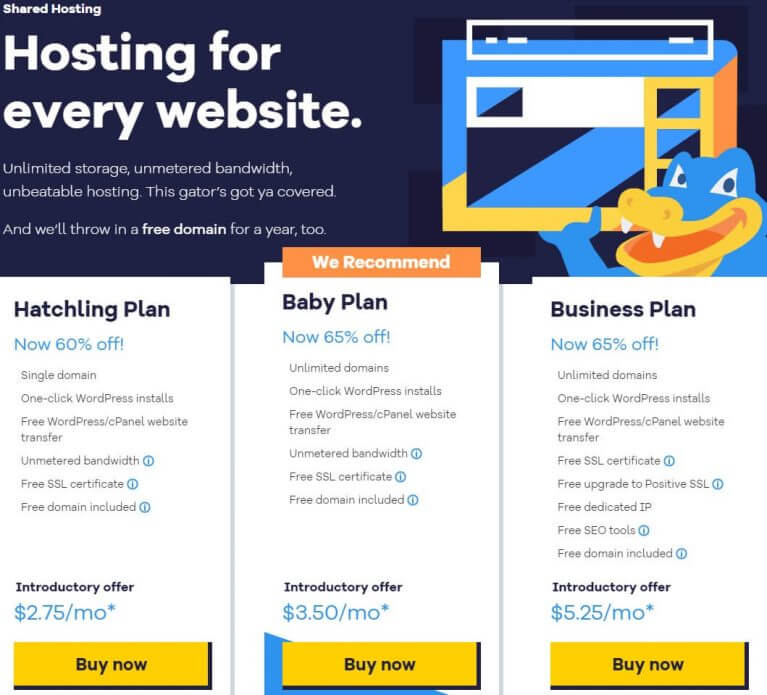This image is a screenshot of a website offering web hosting services, characterized predominately by a white background. The top section, constituting about one-third of the screenshot, is a striking deep navy blue. In the top left corner, small text reads "Shared Hosting." Below this, in a larger white font, is the headline "Hosting for Every Website." Further down, in smaller text, several benefits are listed: "Unlimited Storage, Unmetered Bandwidth, Unbeatable Hosting, This Gator's Got You Covered, and We'll Throw in a Free Domain for a Year Too." 

On the right side of this top section, there is a visually appealing, stylized design of a web page rendered in light blue, yellow, white, peach, and black. This graphic is supported by an illustration of a blue alligator with a yellow mouth and an orange tongue, reinforcing the brand's mascot.

Beneath this header section, the webpage displays three columns detailing different web hosting plans. The leftmost column describes the "Hatchling Plan," now 60% off at a promotional price of $2.75 per month. The central column, highlighted as the recommended option, presents the "Baby Plan," available for an introductory rate of $3.50 per month with a 65% discount. The rightmost column features the "Business Plan," which is also offered at a 65% discount, amounting to an introductory price of $5.25 per month.